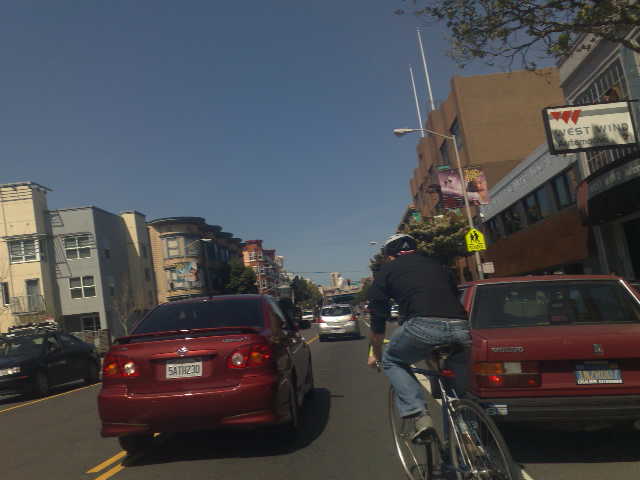This photograph captures the viewpoint from a driver's perspective on a moderately congested street. The thoroughfare features a single lane in each direction, flanked by parked cars on both sides. 

On the left side of the street, there are low-rise buildings that appear to be residential. These structures are grey and beige, standing at about three stories tall, and lined with numerous windows. 

To the right, a bright yellow pedestrian crossing sign prominently displays two walking figures, signaling a designated walkway. Adjacent to the sign are darker beige and brown buildings that resemble storefronts, contrasting with the residential feel of the left side.

In the immediate foreground, a red sedan is visible directly in front of the camera's vantage point. Adding to the dynamic scene, a cyclist is captured cutting directly across this viewpoint. The cyclist is wearing a white helmet, a black long-sleeved shirt, and jeans, navigating through the traffic.

Further ahead in the center of the image, a silver car can be seen on the road. Parked to the right, directly beside where the cyclist is maneuvering, is another red sedan. 

The detailed elements in this photograph combine to create a vivid portrayal of an urban street scene bustling with daily activity.